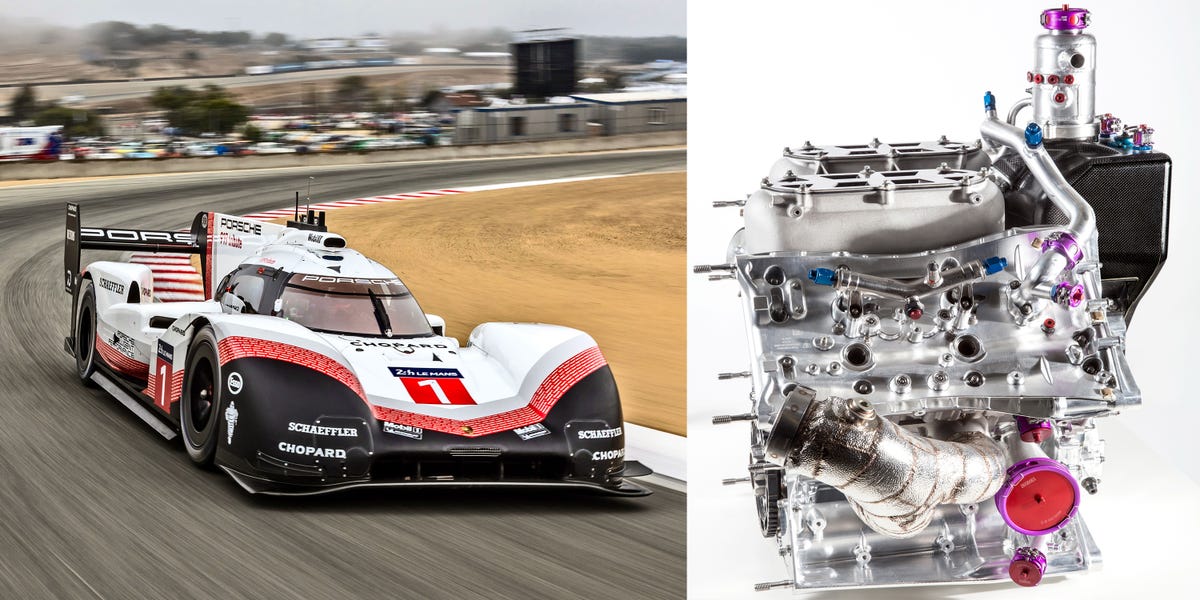The image on the left captures an action-packed scene of a Porsche racing on a track, coming into view towards the camera as it exits a sharp left corner and enters a straightaway. The car is a sleek white and black design, featuring a distinctive red stripe that extends from the front over the side skirts. The car proudly displays the PORSCHE branding on a black spoiler and a black visor over the windshield. Various company advertisements, including Schaefer and Chopard, decorate the vehicle. The track beneath the car is gray with black streaks, bordered by red stripes in some sections. In the background, there is a blurred view of other cars and buildings, hinting at the bustling activity of the racetrack environment.

The image on the right showcases a detailed, silver and chrome-colored engine. This intricate motor is adorned with colorful elements including pink, blue, and red gears, along with black knobs and a prominent red cap at the bottom. A large metal hose is visible on the right side, completing the complex mechanical setup.